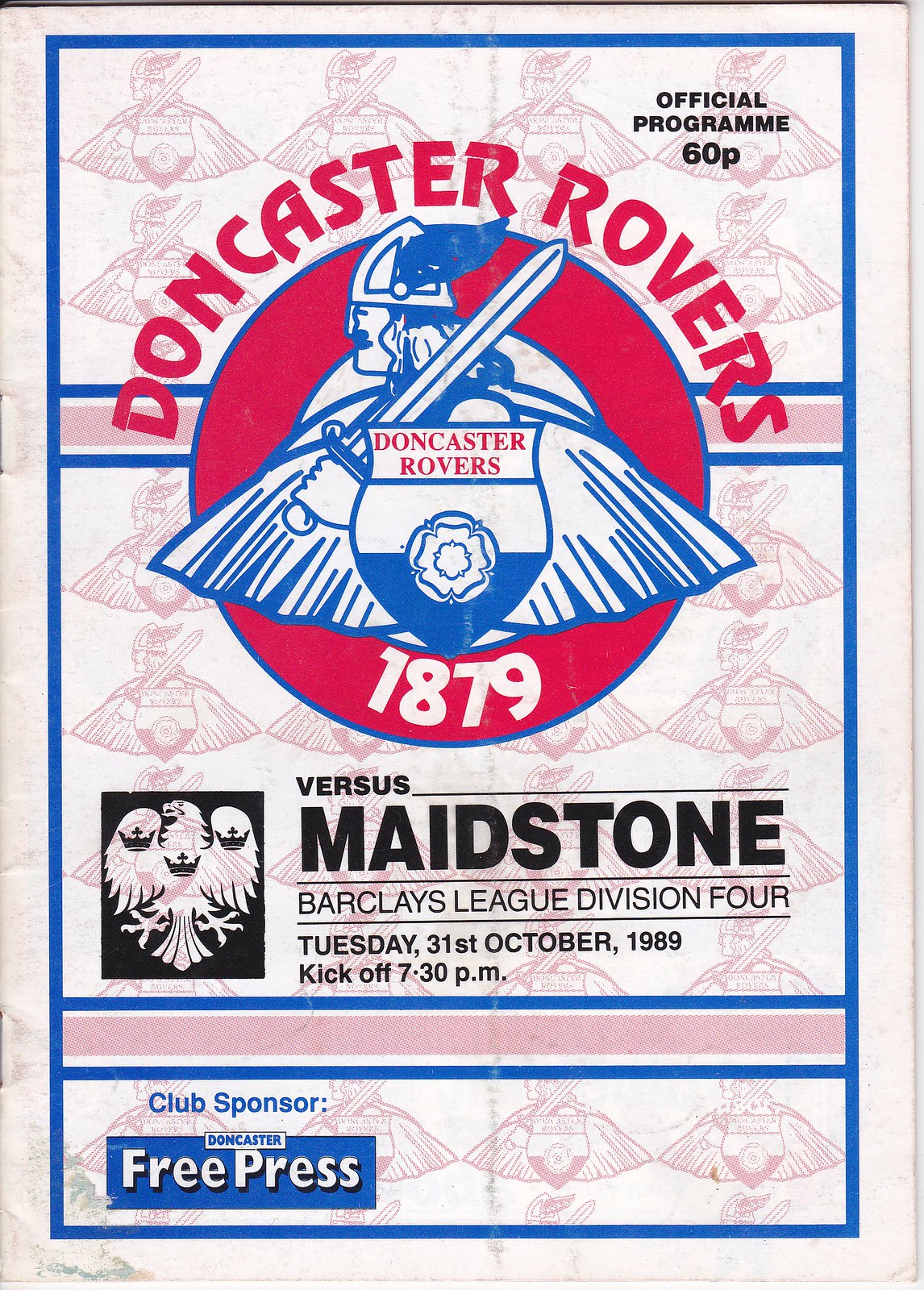The image showcases the cover of an official Doncaster Rovers program, priced at 60 pence. Central to the design is a prominent blue and white Viking holding a sword in his left hand, with "Doncaster Rovers" and "1879" indicating the team's establishment year. The program cover, which features a light red, white, and blue color scheme, also includes the opposing team, Maidstone, with their logo. Details about the match such as "Barclays League Division 4," "Tuesday, 31st October 1989," and "Kickoff, 7:30 PM" are displayed below the Viking emblem. The top right corner marks it as the "Official Program," and at the bottom, it notes the club sponsor, Doncaster Free Press. The program is bordered in white and secured together with two staples on the left side.